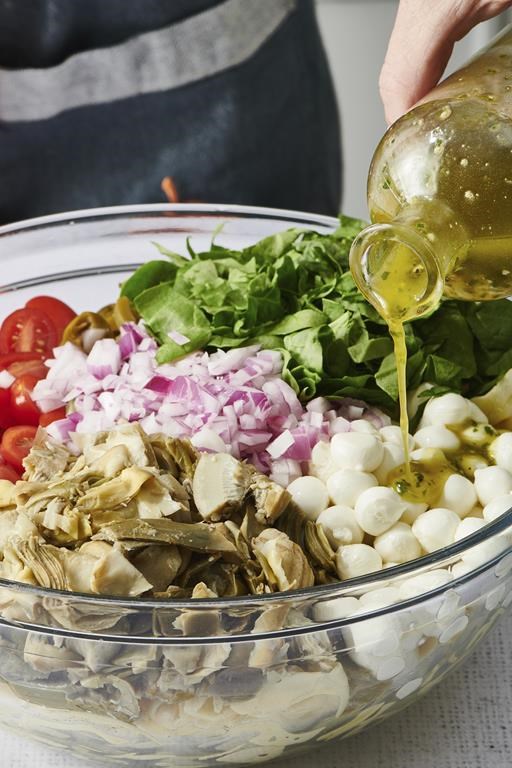In this image, a person wearing a black shirt with a gray stripe pours a dark green, oil-based vinaigrette salad dressing from a glass bottle onto a colorful, vibrant salad. The salad, which is presented in a glass bowl, features an array of fresh ingredients including lettuce leaves, halved cherry tomatoes, red onions, artichokes, and little balls of mozzarella cheese. There also appear to be pieces of chicken or another brownish vegetable, along with possible chickpeas and mushrooms, though the ingredients are somewhat separated into distinct piles within the bowl. The scene is set against a speckled, wooden-textured surface, with the focus on the dressing being drizzled over the ingredients, beginning to meld these varied elements into a delicious and visually appealing dish. The person's white hand, which is the only visible part of them, suggests careful attention to the task at hand, adding the final touch of flavor to this large, healthy salad.